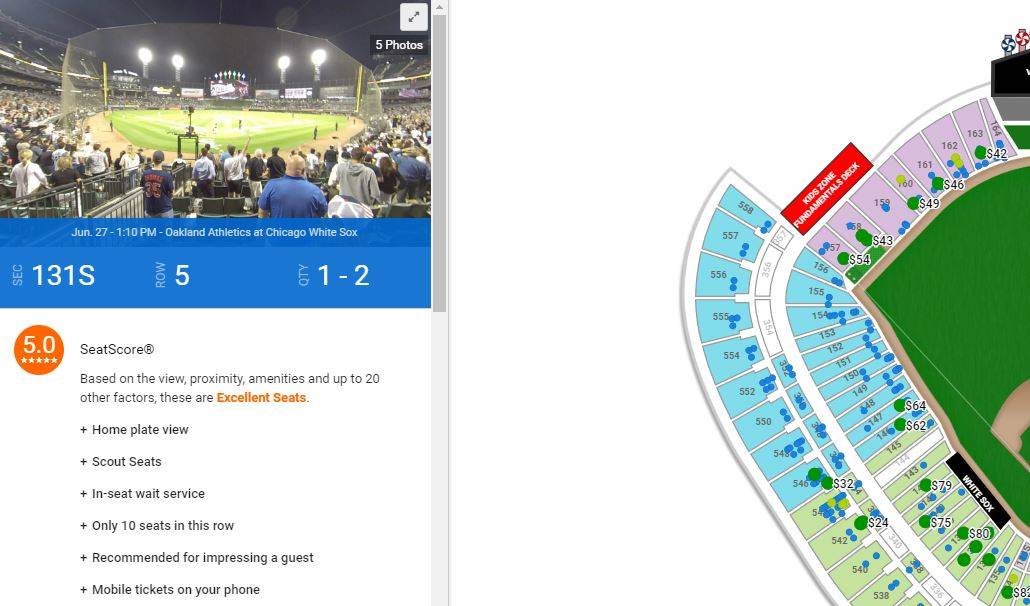The image is divided into two sections. The right section presents a detailed seating plan for a baseball game, indicating ticket prices and seat locations. At the very bottom right, there's a small white box displaying ticket prices: $79, $75, and $80. Above this box and towards the right center, there's a green playing field surrounded by various ticket prices such as $54, $43, $49, $46, and $42. The left of this section highlights the "Kids Zone Fundamentals Deck" in red text, emphasizing it as a special seating area.

On the left section of the image, there's an image of a baseball field accompanied by text indicating "June 27th, 1:10 p.m. - Oakland Athletics at Chicago White Sox." The top right corner mentions "5 photos," referencing additional views or images. This section details specifics about the seats, noted as "Section 131S, Row 5, Quantity 1-2." This likely shows the exact view from these seats. The information below describes a "Seat Score" based on various factors like view, proximity, and amenities, giving these seats a perfect score of 5 out of 5. These seats, identified as "home plate views, scout seats," offer in-seat wait service and have only 10 seats in the entire row. They are recommended for impressing guests and come with mobile ticketing options. However, the price for these seats is not provided in the image.